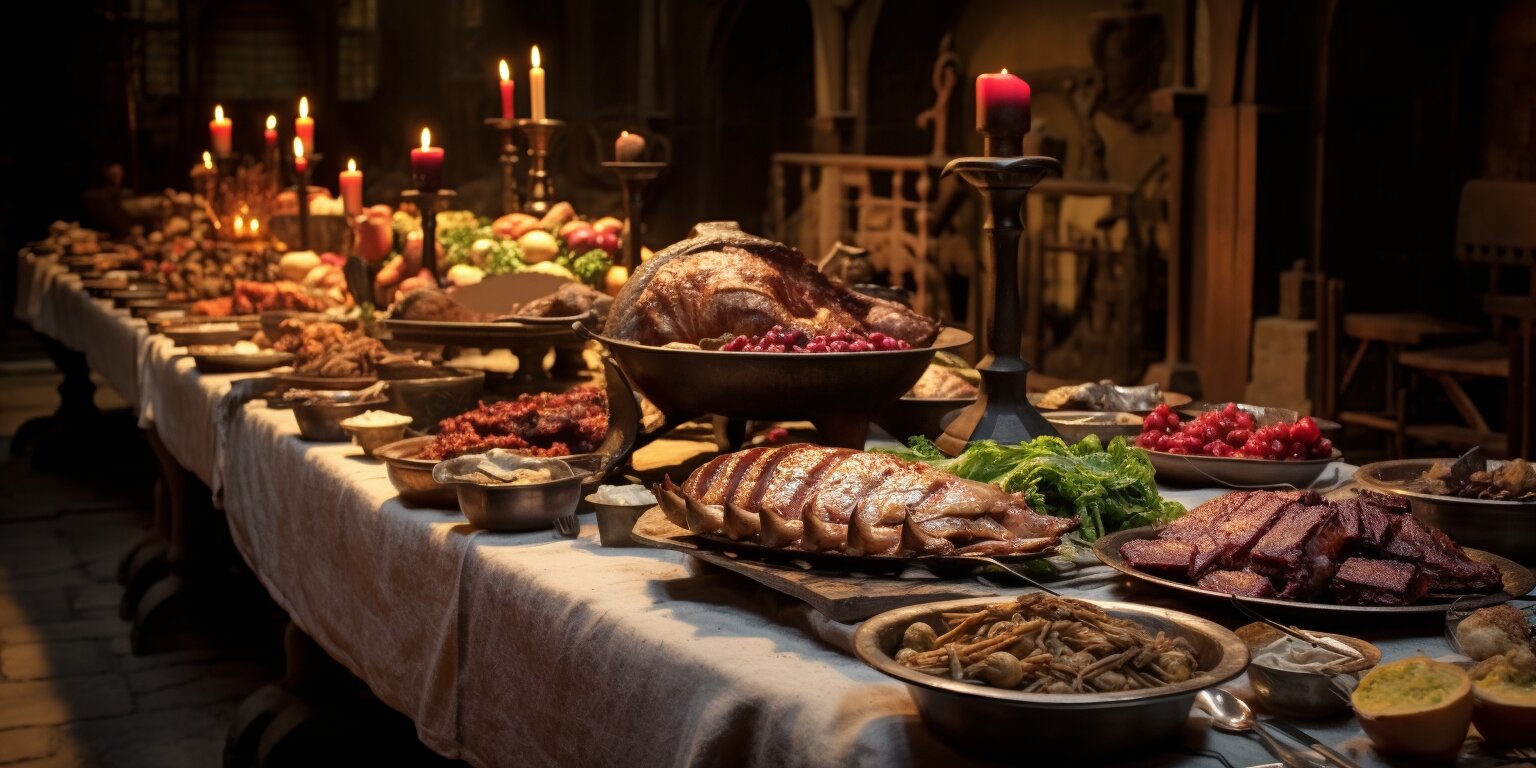This is a horizontally aligned rectangular image depicting a grand medieval banquet setting, resembling a scene from historical times or a medieval-themed movie. The long rectangular table, covered with a white tablecloth, is lavishly adorned with an abundance of food, including large, silver, tin, or lead-like serving plates and bowls filled with an assortment of meats, fruits, and vegetables. In the center of the table, there's an impressive tall round dish featuring what appears to be a roasted chicken or duck, surrounded by small round potatoes. Scattered along the table are other delicacies, such as slices of meat, pieces of bread, lettuce, and cherry tomatoes, accompanied by red berries and whole fruits. The entire setup is well lit by numerous lit candles, including tall candlesticks with both big circular and small cylindrical candles. The background remains quite dark, contrasting the well-lit table, and features intricate wood-carved archways and woodwork, somewhat resembling wrought iron made from wood. The floor in the image is ambiguous, appearing either as hand-cut wooden slats or stone tiles set with mortar, adding to the rustic and historical ambiance of the scene.